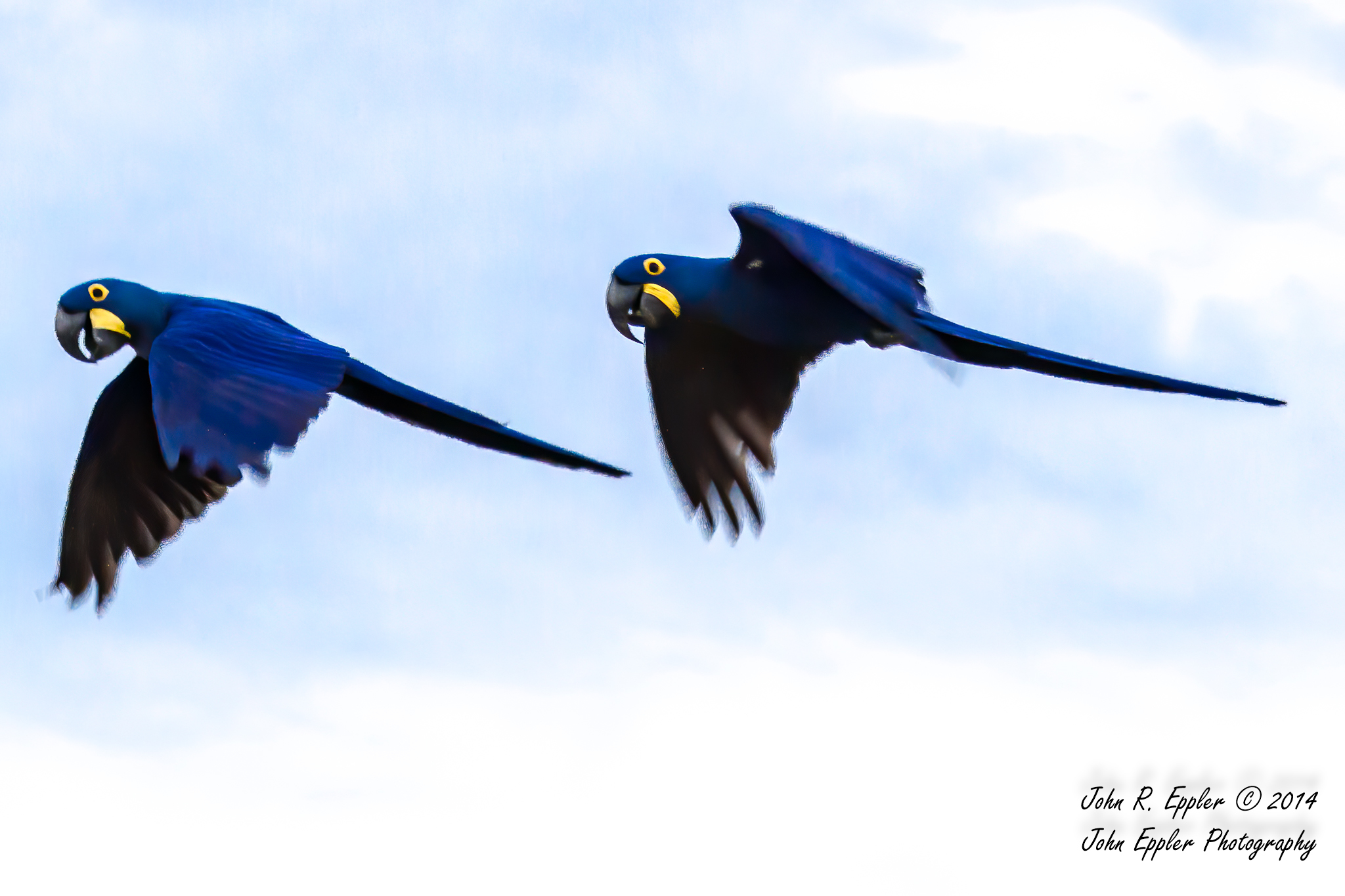This horizontal photograph captures two striking dark blue birds in mid-flight, both oriented towards the left side of the image. The birds, resembling parrots or possibly toucans, exhibit vibrant blue feathers with a slightly darker shade on their undersides. They have prominent black beaks, yellow eyes with black centers, and a distinctive yellow ring at the base of their beaks. The birds are flying in unison, with their wings spread downward and their tail feathers extended behind them. The background showcases a serene, pastel blue sky accompanied by faint, diffuse white clouds. In the lower right corner, black text reads "John R. Epler © 2014, John Epler Photography," indicating the artist's signature and copyright information. The image has a realistic yet perhaps slightly enhanced or edited aesthetic, adding to its visual appeal.